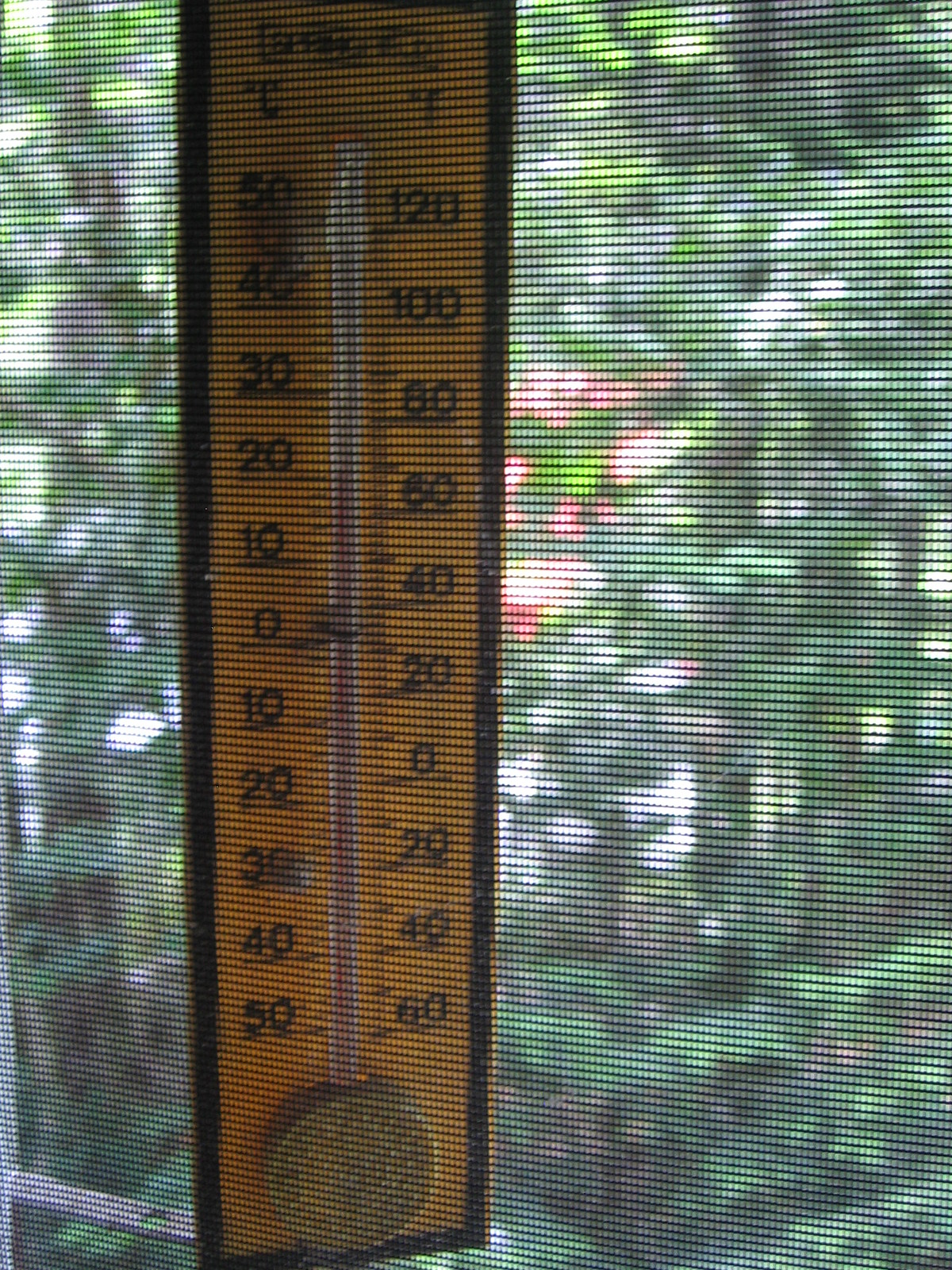This color photograph, taken indoors, captures an intricate view of a screen door. The wire screen clearly delineates the scene, providing a detailed glimpse into the vibrant outdoor setting beyond. Through the mesh, one can see lush greenery, with trees, plants, and grass populating the space. Adding a burst of color, some pink flowers are in full bloom, enhancing the natural beauty of the garden.

Attached to the inside of the screen door is a distinctive brown thermometer. The thermometer, which contains mercury, prominently displays a red line indicating the temperature. Though the exact temperature reading is indistinct, it appears to hover around 65 to 70 degrees Fahrenheit. The thermometer has a fabric-like appearance, bordered in black, and hangs securely against the screen’s intricate mesh.

The thermometer's casing houses the red mercury column and features temperature markings in black. The left side of the thermometer is labeled with Celsius, ranging from 30 degrees down to -50 degrees, while the right side is marked in Fahrenheit, from 120 degrees down to -60 degrees. This detailed depiction encapsulates both the functionality and aesthetic charm of the scene, offering a window into a serene and lively outdoor environment.